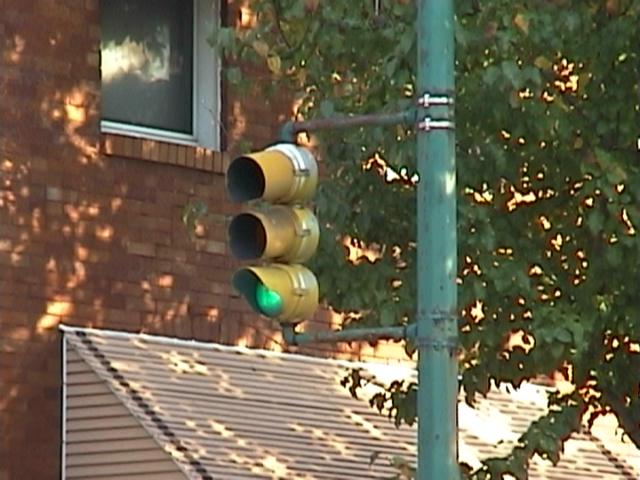In the bright sunlight of a clear day, a traffic light is mounted on a green metal pole in front of a red brick building that stands at least two stories high. The traffic light, encased in a goldish metal cone, displays a green light while the other two lights remain dark. Behind the pole, the top leaves of a tree are visible, providing a contrast of greenery against the man-made structures. Adjacent to the traffic light, the red brick building features a single visible window. Below this window, several feet down, there's a white siding canopy extending from the building, partially illuminated by dappled sunlight and shadows, adding texture and depth to the scene.